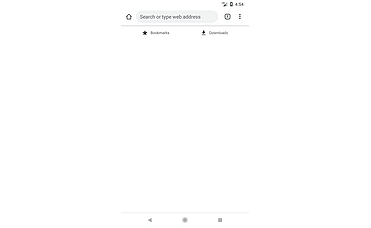This detailed caption describes an intricate miniature screenshot from what appears to be a mobile device or a small desktop window. 

---

The image captures a tiny screenshot, likely from a mobile device or a minimized desktop window, displaying a primarily white background. At the screen’s top right corner, small Wi-Fi and battery icons are visible, with the time reading "4:54" adjacent to them. 

Along the top, the title bar includes a house icon next to a search bar, which contains a web address reference. To the right of the search bar, an additional icon and a three-dot menu are present. A thin line separates this header section from the content below. 

Within the main body of the window, two distinct areas of information are separated by ample white space. Each section contains an icon paired with some textual information. 

At the very bottom of the screenshot, another thin dividing line is observable, beneath which three more icons are aligned horizontally.

---

This caption ensures a clear and comprehensive description of the visual elements and layout presented in the miniature screenshot.